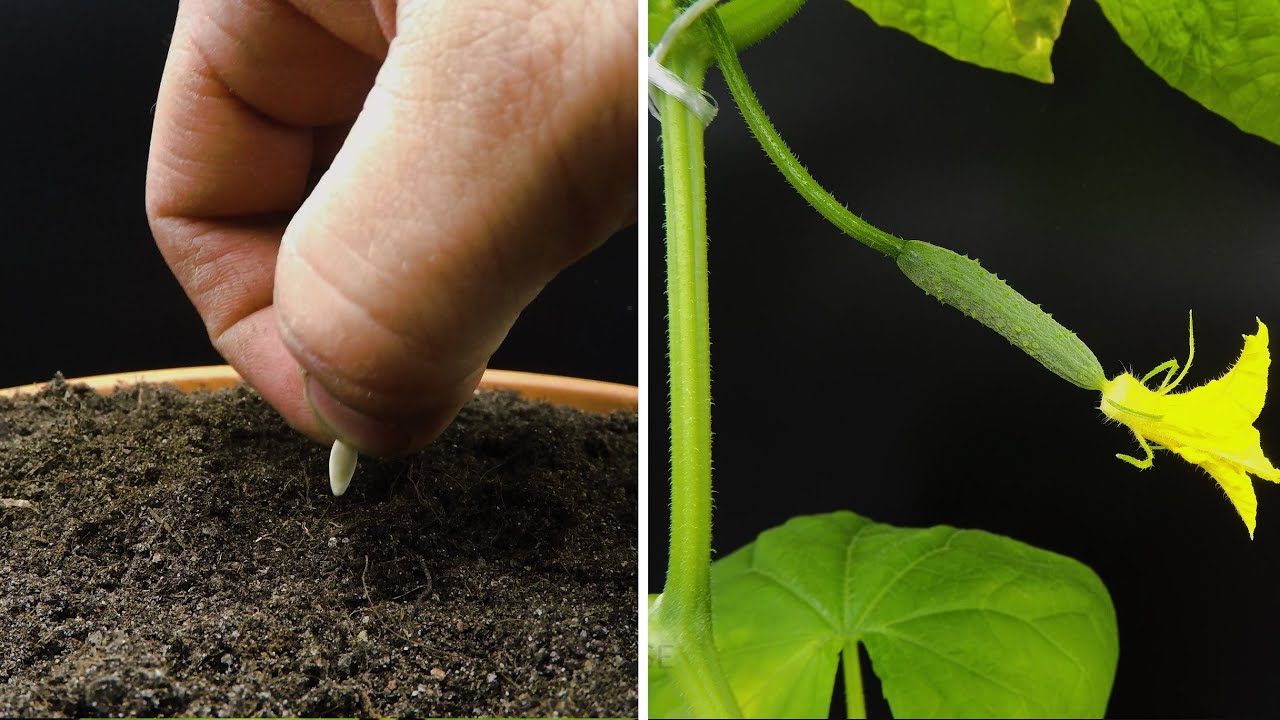In a split-image collage, the left side shows a close-up of a hand with two fingers delicately placing a small white seed into the rich, dark soil of a pot, suggesting the initial act of planting. The right side contrasts this with the vibrant growth resulting from that seed—a short-stemmed green cucumber plant with detailed leaves, prominently displaying a small, bright yellow flower trailing to the right. Both parts of the image are set against a striking black backdrop, emphasizing the transformation from seed to bloom. The details of the soil, the hand, the seed, the plant, the leaves, and the flower collectively illustrate the growth process from inception to the early stages of fruition.